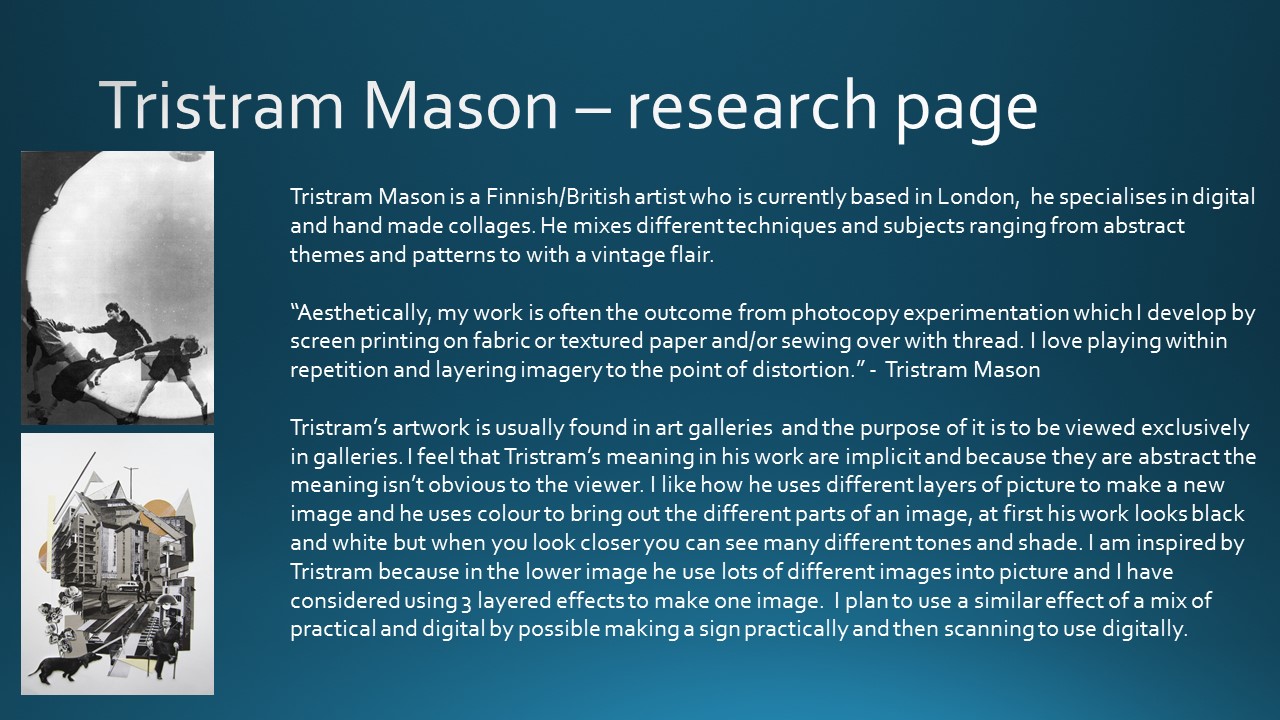The research page of Finnish-British artist Tristram Mason, currently based in London, features a blue background topped with the title "Tristram Mason Research Page" in white text. Below, it introduces Mason as a specialist in digital and handmade collages, blending various techniques to create pieces that range from abstract themes and patterns to those with a vintage flair. His work is characterized by photocopy experimentation, often developed through screen printing on fabric or textured paper, and sewing with thread. Mason enjoys playing with repetition and layering imagery to the point of distortion, resulting in multi-layered, detailed works that might initially appear black and white but reveal numerous tones and shades upon closer inspection. His art, meant to be viewed exclusively in galleries, uses color to highlight different parts of an image, making the implicit meanings within his abstract pieces more intriguing. Accompanying the text on the left-hand side are two enigmatic square photos that enhance the visual appeal of the page.